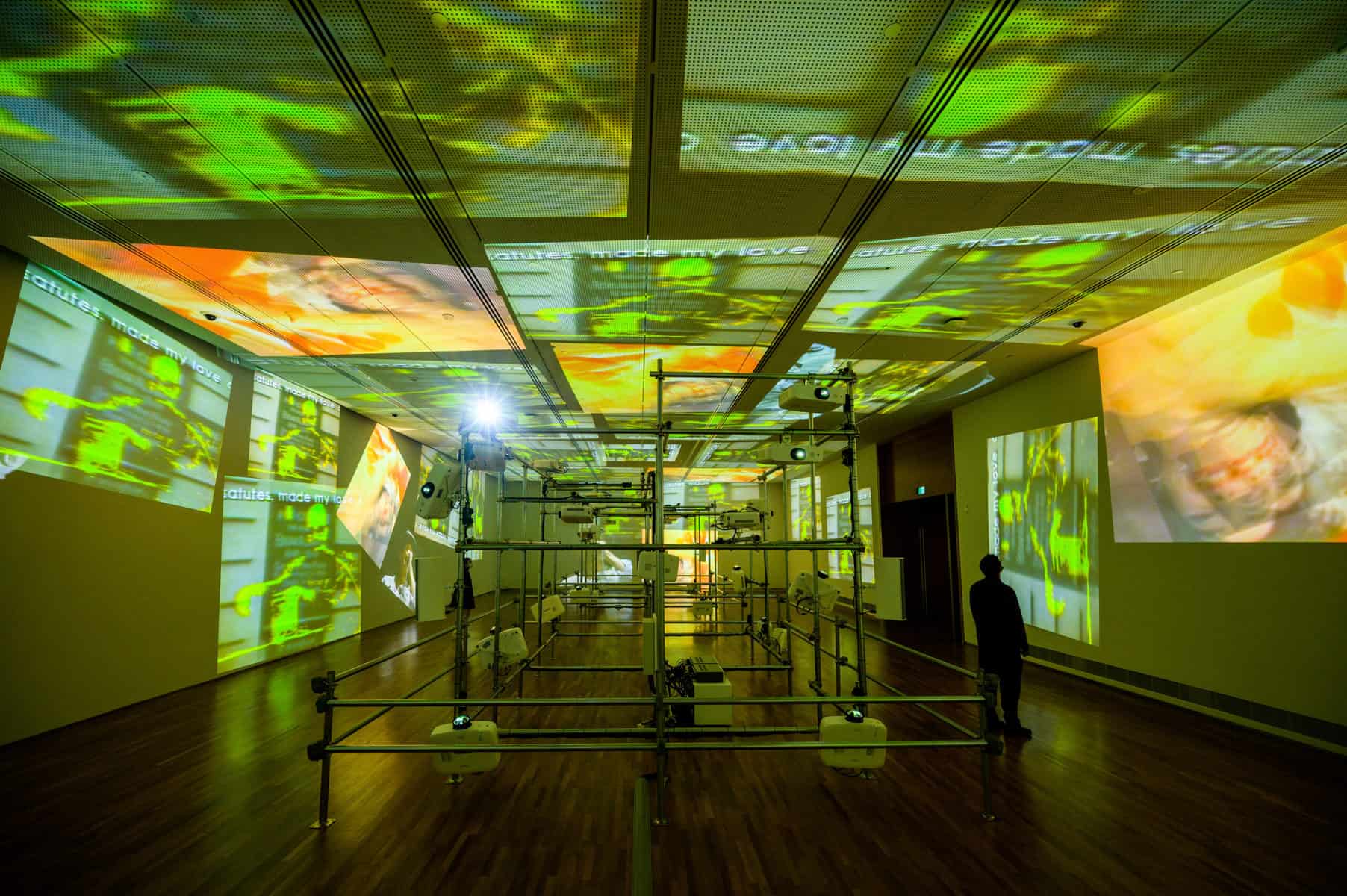The scene depicts a long, expansive room with polished wooden floors, immersed in darkness with a subdued, ambient light emanating from projections on the walls and ceiling. The projections display a variety of vivid and surreal images, such as a neon green figure seated in a chair and an orange-hued woman with a rapidly moving face, creating multiple overlapping impressions complete with striking red lipstick. Steel scaffolding structures run through the center of the room, adorned with projectors facing different directions, casting these images onto the surrounding surfaces. A single person stands on the right side of the room, gazing upward at the ceiling projections. A door is noticeable midway along the right wall, subtly integrated into the intricate visual environment.